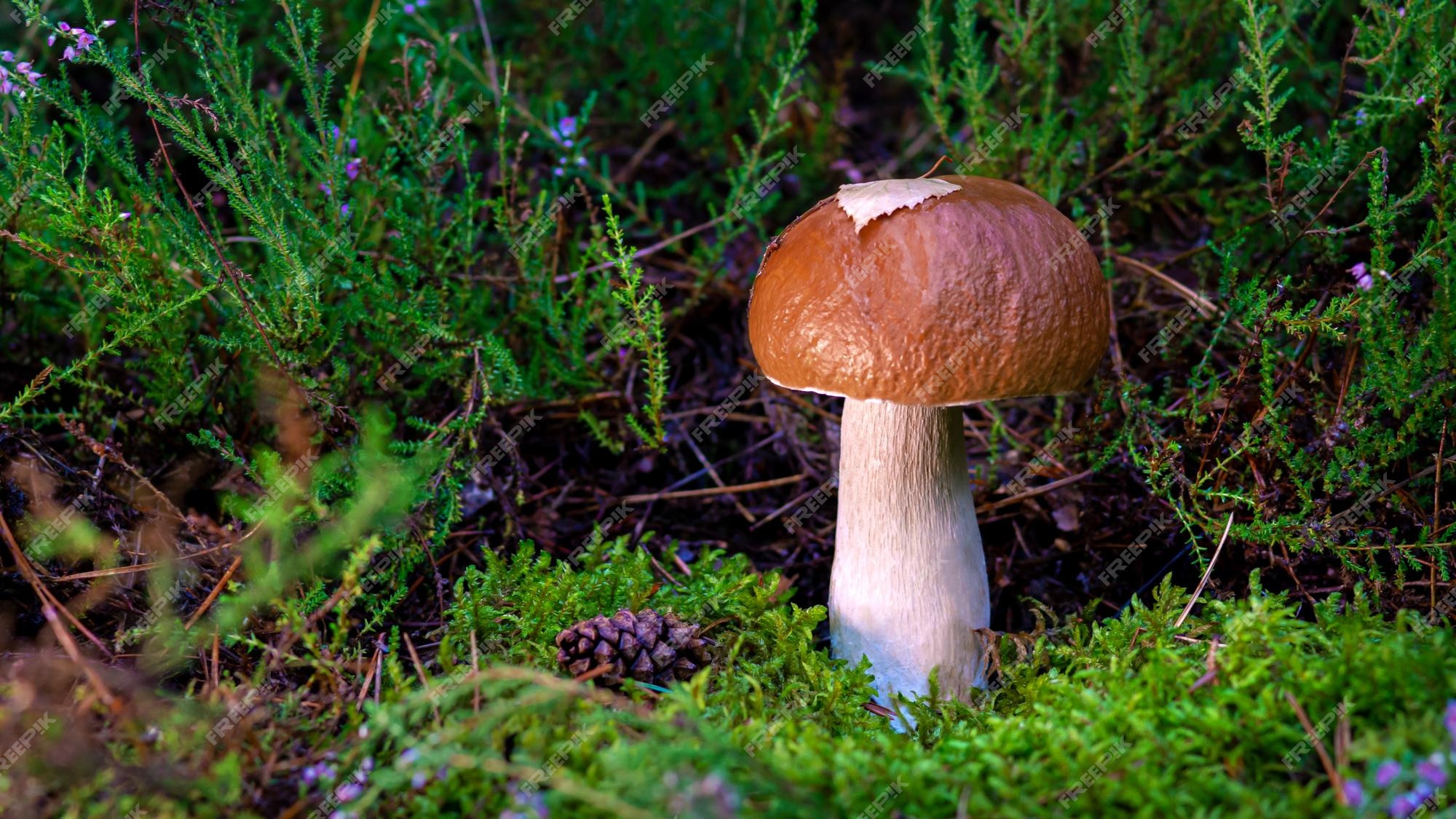A vibrant, detailed close-up photograph captures a striking mushroom with a shiny brown cap, crowned by a baby leaf. The mushroom's thick white stem stands proudly from a bed of lush, green moss-like plants. Surrounding the mushroom are slender, needle-like green leaves and a miniature pine cone nestled at the forest floor. The scene is softly lit, evoking a surreal, fairy tale ambiance. The mushroom dominates the image, seemingly emerging from a ferny, woodsy ground. There are subtle touches of additional flora, including purple-hued plants and some dark grass, contributing to the overall enchanting and pristine forest setting on what appears to be a beautiful day.